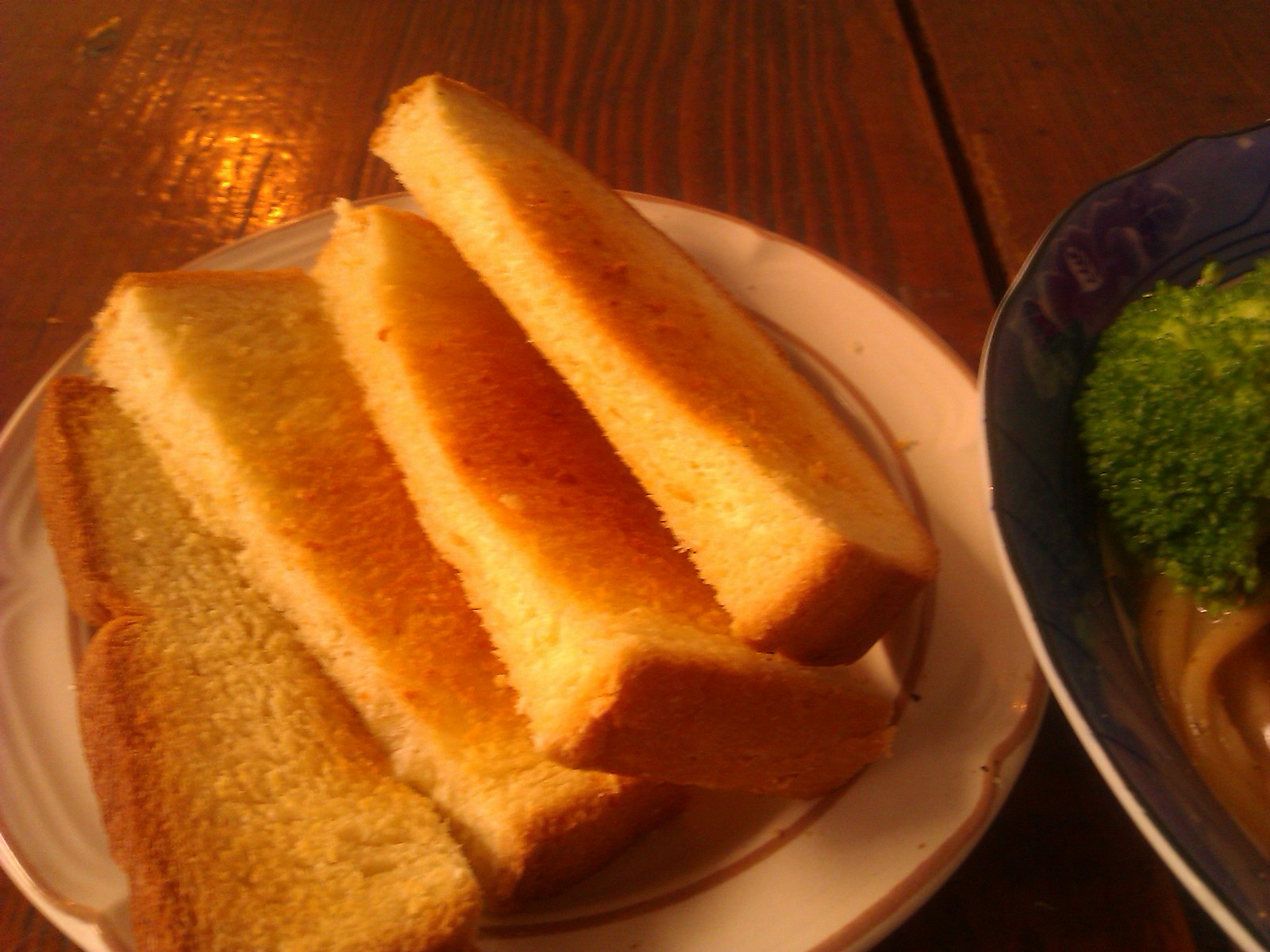This photograph, likely taken in a kitchen or dining area, features a meal set on a dark wooden table with a slatted design. The focal point is a white ceramic plate, round in shape with scalloped edges and a golden trim, holding four slices of toasted sourdough bread. To the right of the plate sits a blue bowl with a white trim, containing a dish of noodles and broccoli florets, possibly seasoned with spices or condiments. The lighting in the room is dim, casting a subtle reflection on the table's surface, especially noticeable in the upper left corner of the image.